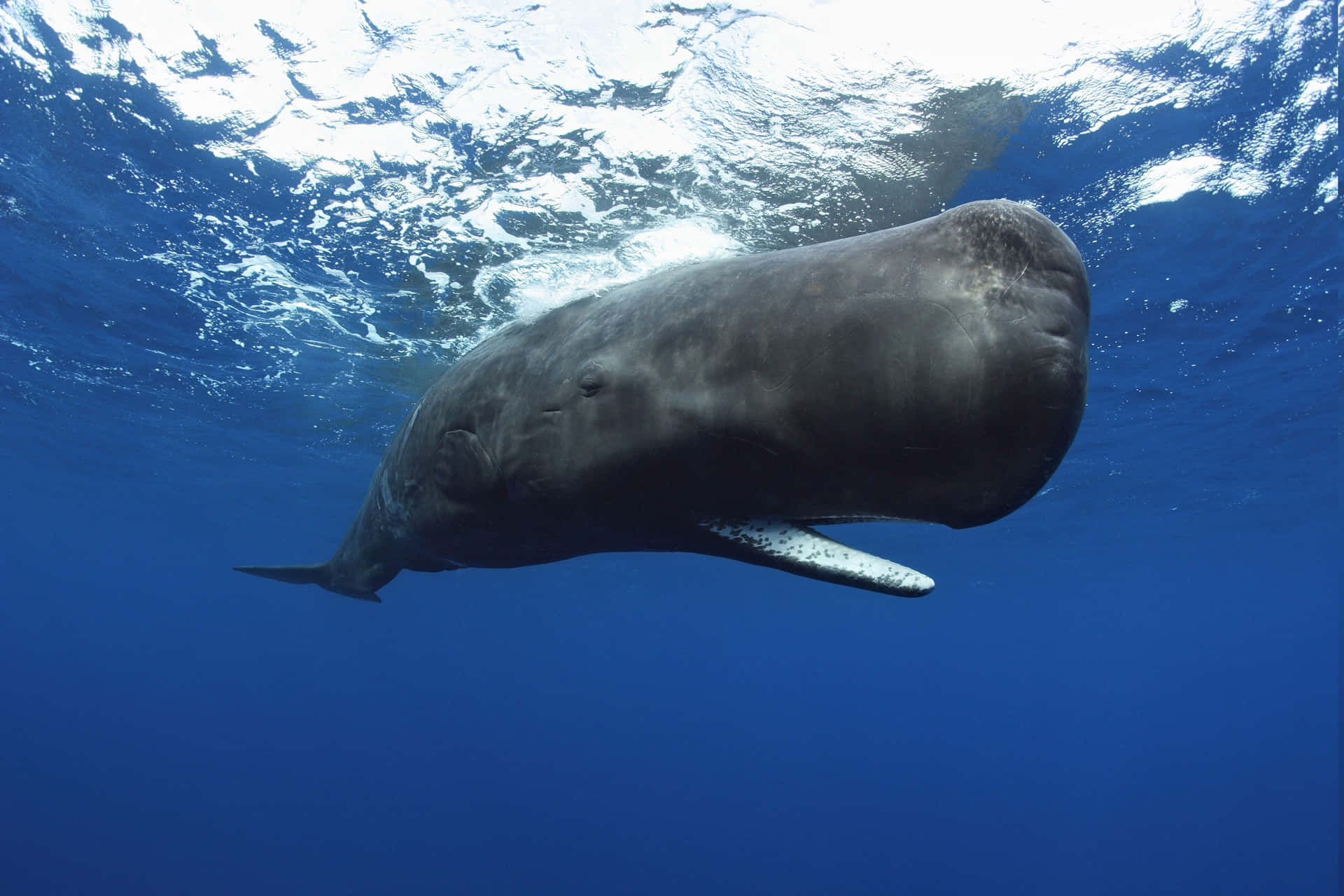This detailed underwater photograph showcases a large, dark gray whale, possibly a sperm whale, near the surface of the ocean. The whale dominates the center of the image, its enormous, block-shaped head with rounded corners facing the camera. The whale's eye is a small slit, giving the impression that it is closed. The mouth is partially open, revealing a whitish interior speckled with black spots. The whale's skin is smooth and mostly gray with some silvery shadings. Toward the top of the image, sunlight beams through the water, creating a clear, light blue surface marred with white, foamy waves and bubbles. The water beneath the whale is a deep, clear blue, and no other marine life is visible. The whale's long body tapers off to a smaller fin on the side and a distant tail extending to the left. Overall, the scene captures the serene isolation of this magnificent creature in the vast ocean.